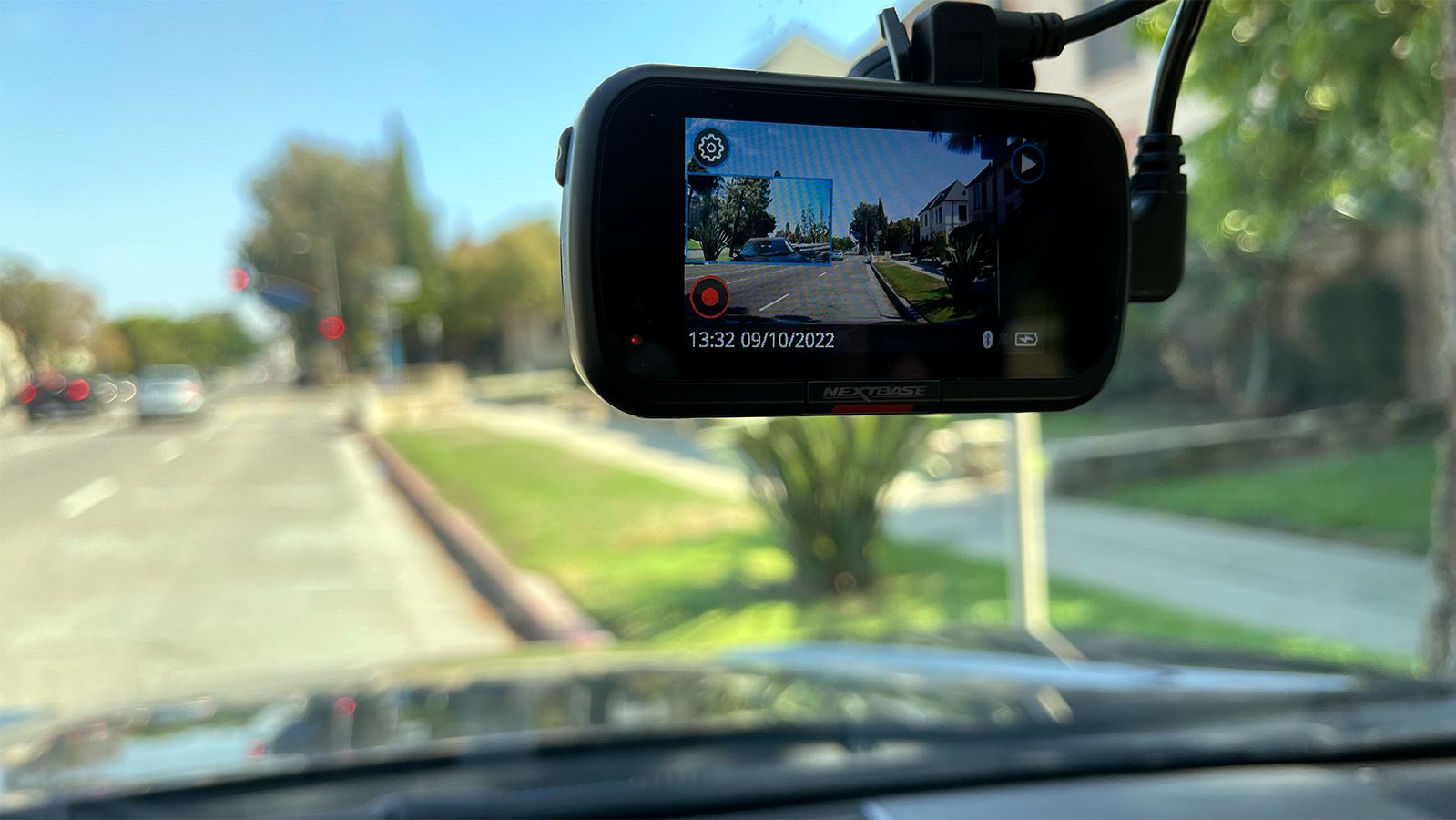The image captures a scene from inside a car, looking outward through the windshield. The entire view outside, including the road, sidewalk, houses, and trees, is blurred, providing a somewhat indistinct background. In the upper left corner of the image, there is a clear blue sky and visible traffic lights with a red signal, along with a couple of cars on the street. The car hood at the bottom of the image also appears blurry.

The main focus of the image is a black rectangular device, likely a rearview camera or GPS navigator, positioned slightly to the upper middle-right side of the frame. This device displays an image that seems to show the rear view of the car or the road ahead, with what could be an accident scene in the feed. It is connected by black cords leading upwards and off the top right of the image.

The screen of this device includes several icons: a white icon at the top left, a red icon at the bottom left, and another white icon with an arrow at the top right. There are additional white icons at the bottom right. The screen also features a date and time stamp in white print at the lower left corner, showing "13:32 09/10/2022."

In the out-of-focus background, the image also shows more trees, buildings, and a grassy median next to the sidewalk on the right side, creating a typical urban or suburban street scene.